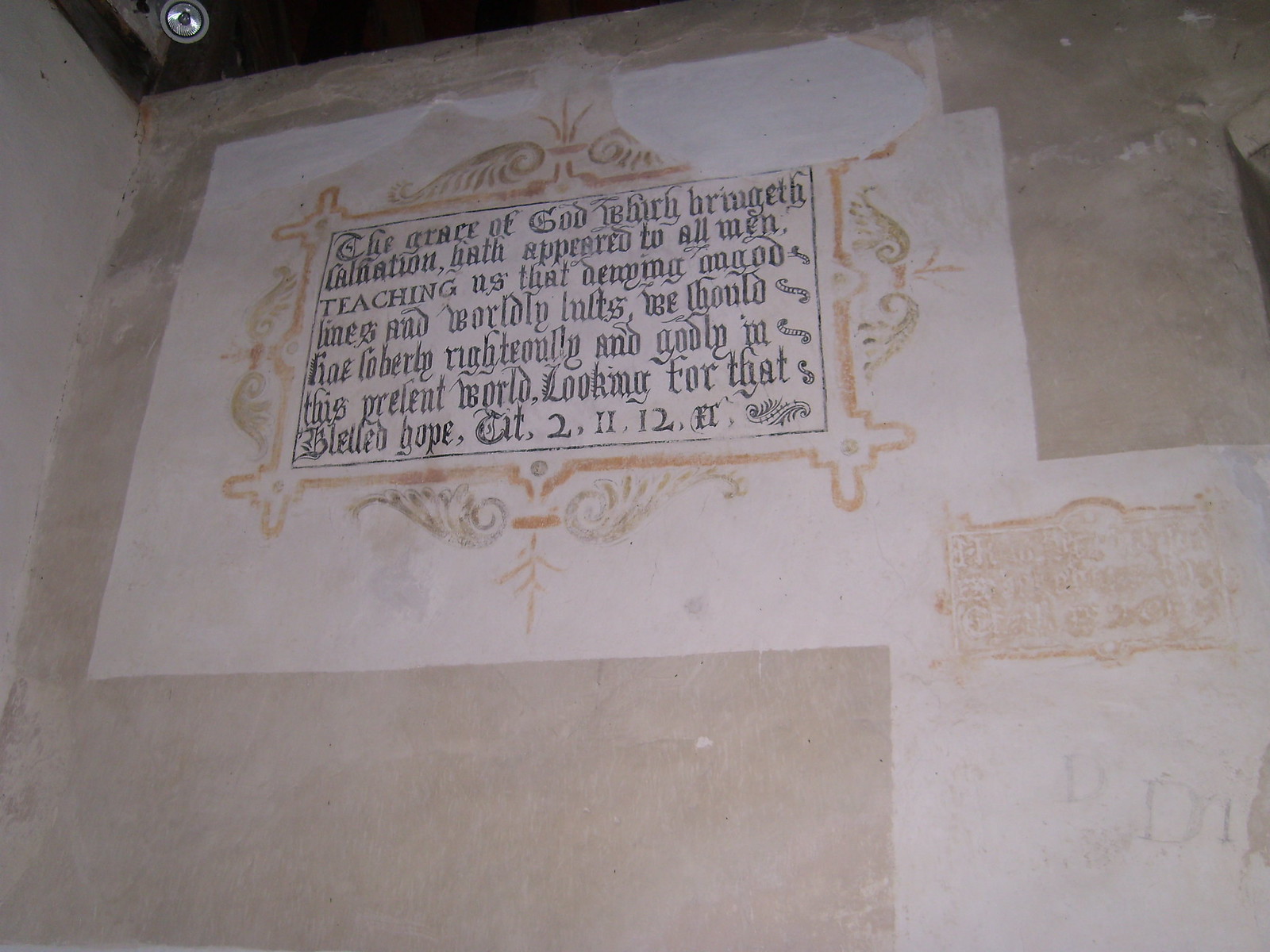This photograph captures a low-angle view of a beige stone or concrete wall, possibly inside a building, as there is a modern light fixture mounted at the top. The wall features two sections painted in a drab white color with ornate gold-colored framing. Inside the frames, there are narrow black borders surrounding an area of similarly white background. The frames enclose very old-style, ornate black text that appears to be a biblical verse. The text is difficult to decipher due to its elaborate typography, but excerpts read: "The grace of God hereby bringeth hath appeared to all men teaching us that denying lines and worldly wants be hold." Additionally, there is a date at the bottom of the text that reads "2-11-12." The overall worn appearance makes the text blend seamlessly with the wall, giving the impression that it is an integrated part of the structure rather than an attachment.